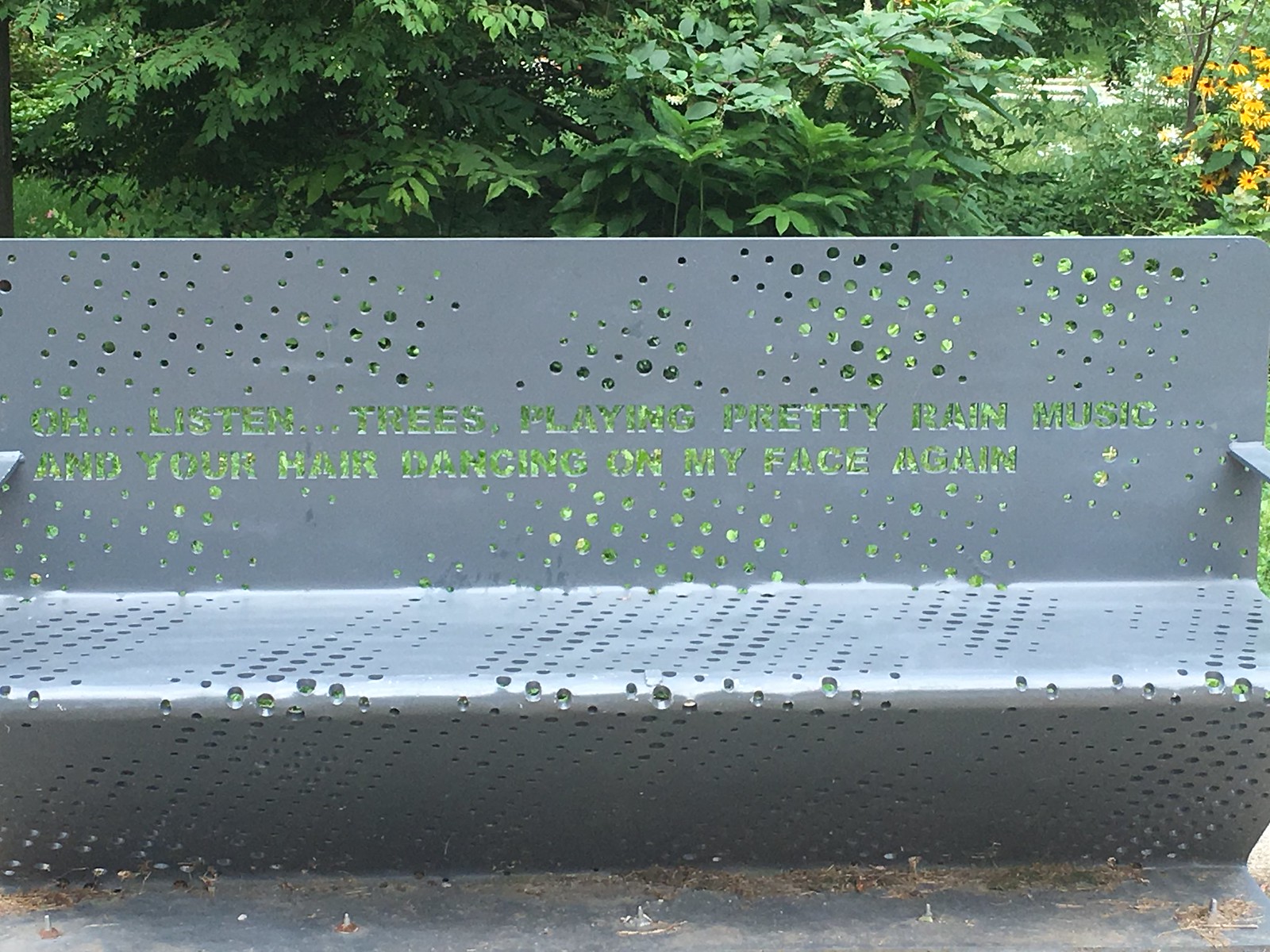This photograph showcases a sturdy gray metal bench, intricately designed with evenly spaced holes drilled in rows across its surface. The backrest of the bench features a poetic inscription that reads, "Oh, listen trees, playing pretty rain music, and your hair dancing on my face again," although the text is somewhat obscured by the lush greenery in the background. The armrest is partly visible on the right side, hinting at the bench's solid, single-piece construction. Surrounding the bench is a verdant array of foliage, including dense green leaves, trees, bushes, ferns, and a splash of vibrant yellow daffodils. There are also black-eyed Susans and daisy-like flowers adding a touch of brightness to this serene park setting.